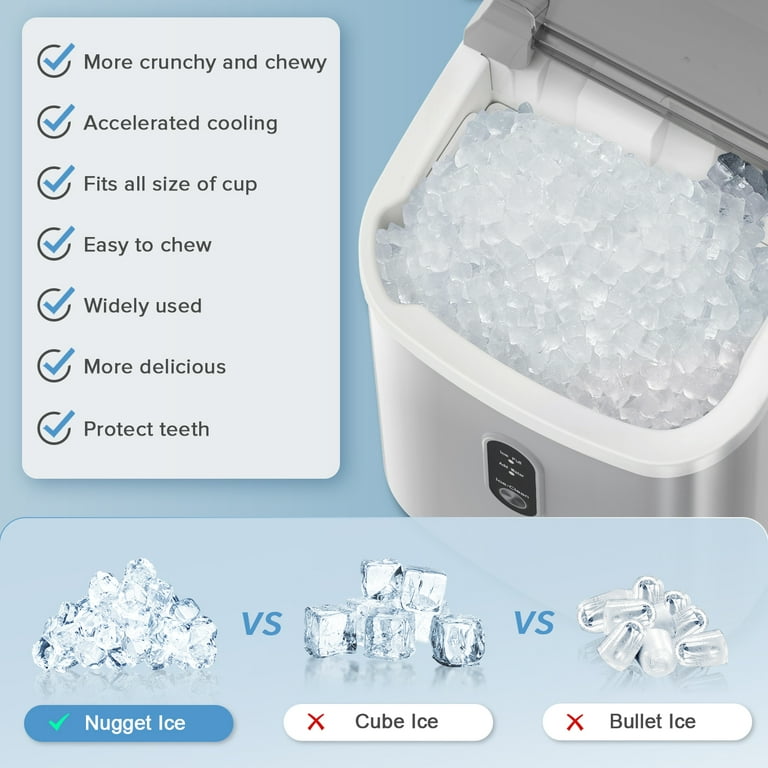The image is an advertisement for a countertop ice maker designed to produce nugget ice, set against a cool, sky-blue background. The close-up of the machine shows its open dark gray lid, revealing a white interior full of nugget ice. The exterior appears to be brushed nickel or stainless steel. To the left of the ice maker, a checklist in a light gray box details the benefits of nugget ice, contrasting against the darker blue. The list highlights features like accelerated cooling, fitting all cup sizes, easy chewability, and dental protection. At the bottom of the image, a comparison chart presents nugget ice as superior, marked with green checks, against cube ice and bullet ice, which are marked with red Xs. The ad emphasizes that nugget ice is the best choice for teeth-friendly, crunchy, and chewable ice.